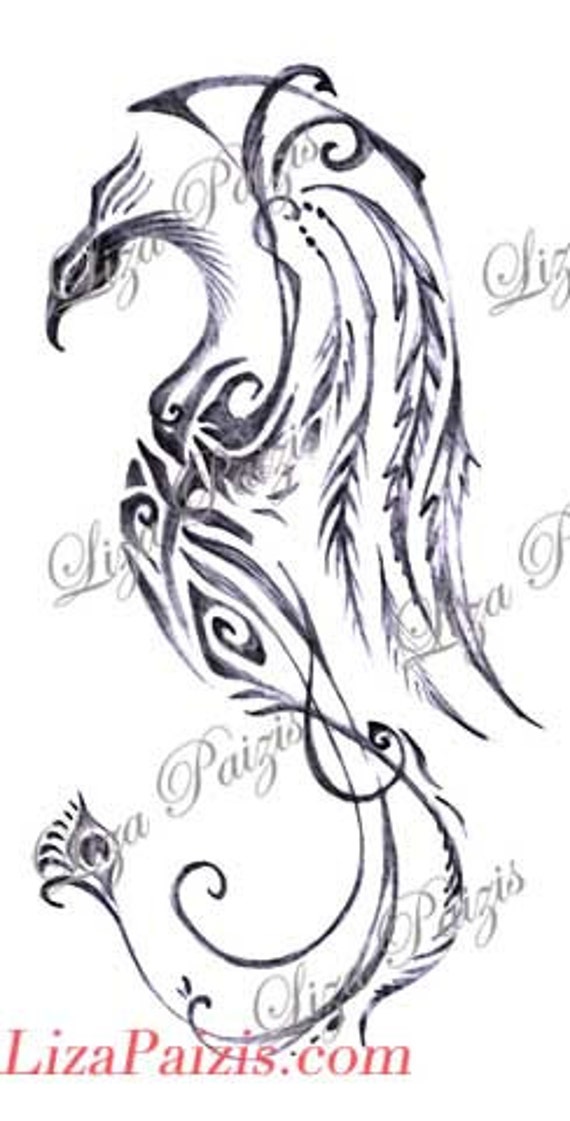The black-and-white hand-drawn artwork depicts a stylized bird, possibly a dragon, phoenix, or peacock, featuring a slender, narrow head and prominent wings extending the length of its body, with no visible legs. The overall design has traditional tattoo-style accents and detailed ink work, suggesting it could be a tattoo template. The bird is positioned with its head and beak in the upper left of the image. At the bottom of the image, in red text, is the artist's website, "LizaPaizis.com" (spelled L-I-Z-A-P-A-I-Z-I-S.com). Additionally, the image contains a watermark of the website's name, indicating ownership and likely protection against unauthorized use.